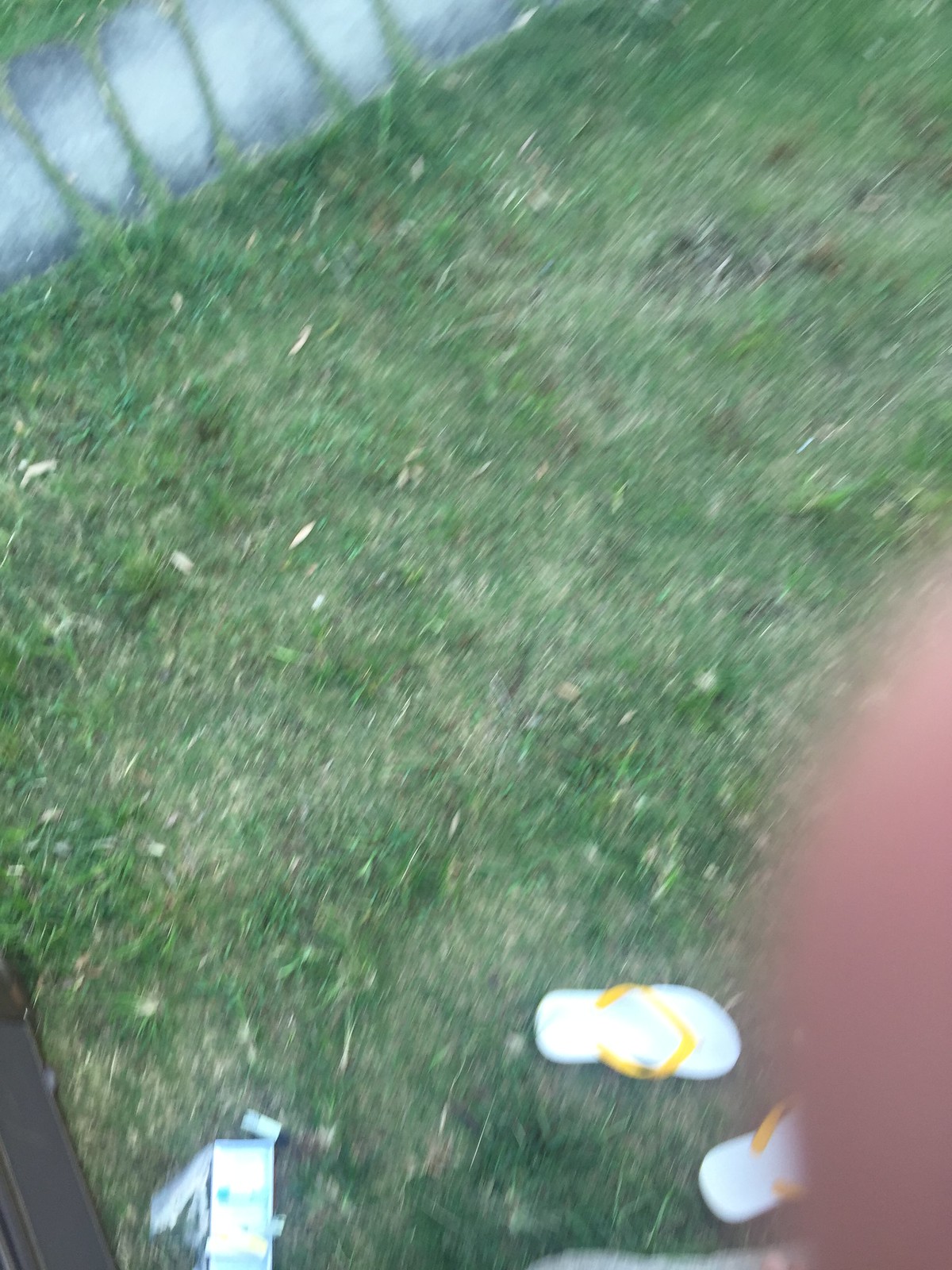This seemingly accidental mobile phone photo captures an aerial view of the ground, featuring an array of elements that tell an intriguing, casual story. The unkempt grass, characterized by various types of blades, dominates the scene, interspersed with small stones that likely outline a flowerbed or walkway near the top of the frame. On the bottom right, a pair of white flip-flops with yellow straps lies haphazardly, with an unidentified object dropped just to their left. A finger partially obstructs the bottom right corner, adding a candid, off-guard feel to the photograph. This snapshot might suggest someone preparing to enter a pool, given the relaxed, informal subject matter and angle.